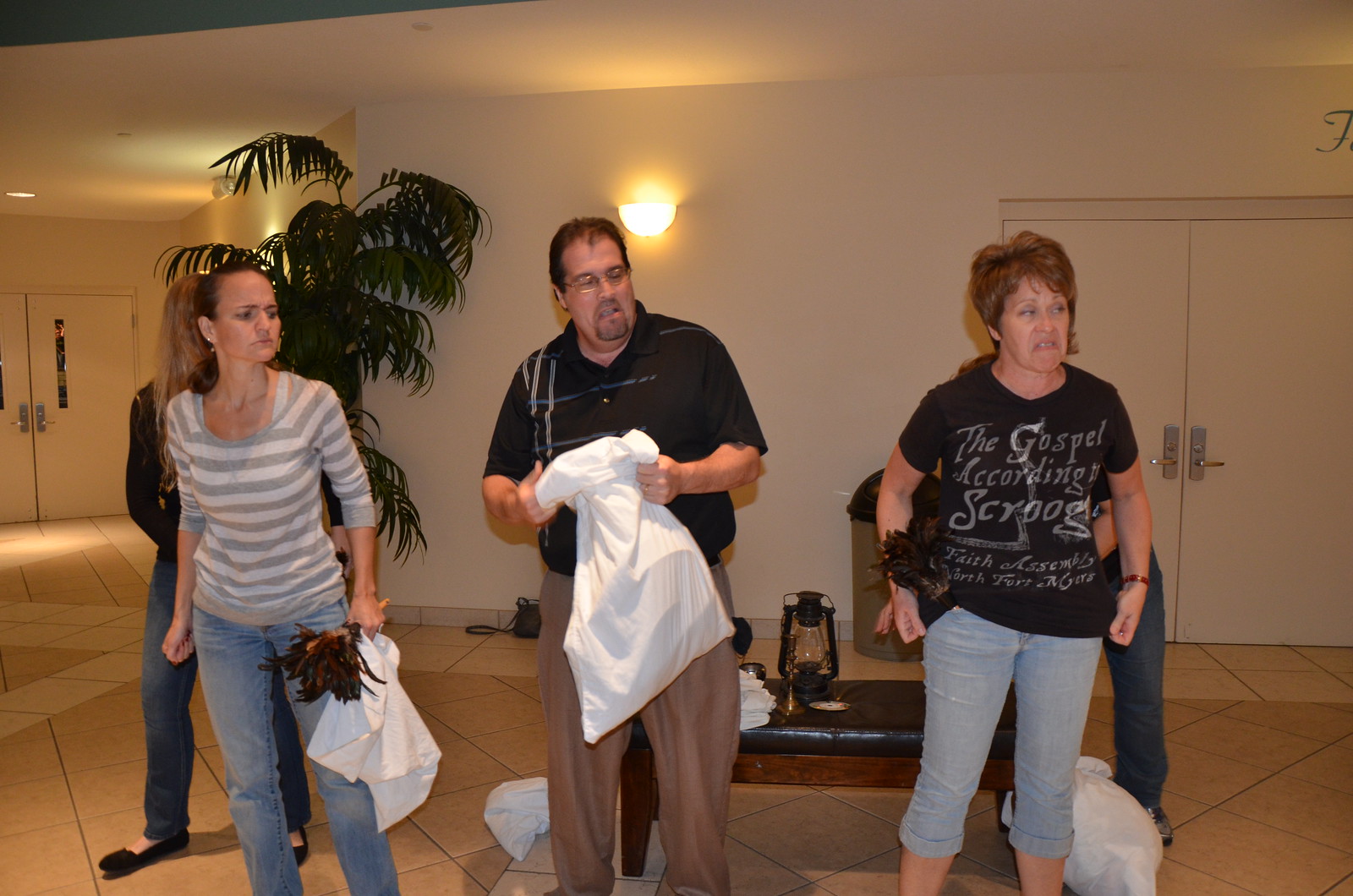In a well-lit room with white walls and double doors on either side, three individuals stand at the forefront, glaring with palpable anger and disgust toward something off-screen to the right. From left to right, the group consists of a teenage girl, an older man, and a woman who appears to be his wife. The teenage girl on the left sports a gray and white striped sweater and blue jeans, her hair tied back in a ponytail. In her hand, she holds a white pillowcase with a brown duster and some white cloth. The man in the center, who wears a black button-up shirt with white stripes and baggy brown pants, clutches a similar white pillowcase that appears to be filled with something. To his right, the woman has short brown hair and wears a black shirt with the text "The Gospel According to Scrooge" partially visible, along with blue jeans that end at her knees. Her hands are by her sides, slightly clenched into fists, emphasizing her grimace. In the background, another figure with blonde hair can be seen partially obscured, wearing a black shirt and blue jeans. A large plant and a lantern on a chair further add to the room's decor. This scene of tension and hostility is set against the backdrop of what seems to be a living area or ballroom, marked by the distinct tile flooring.